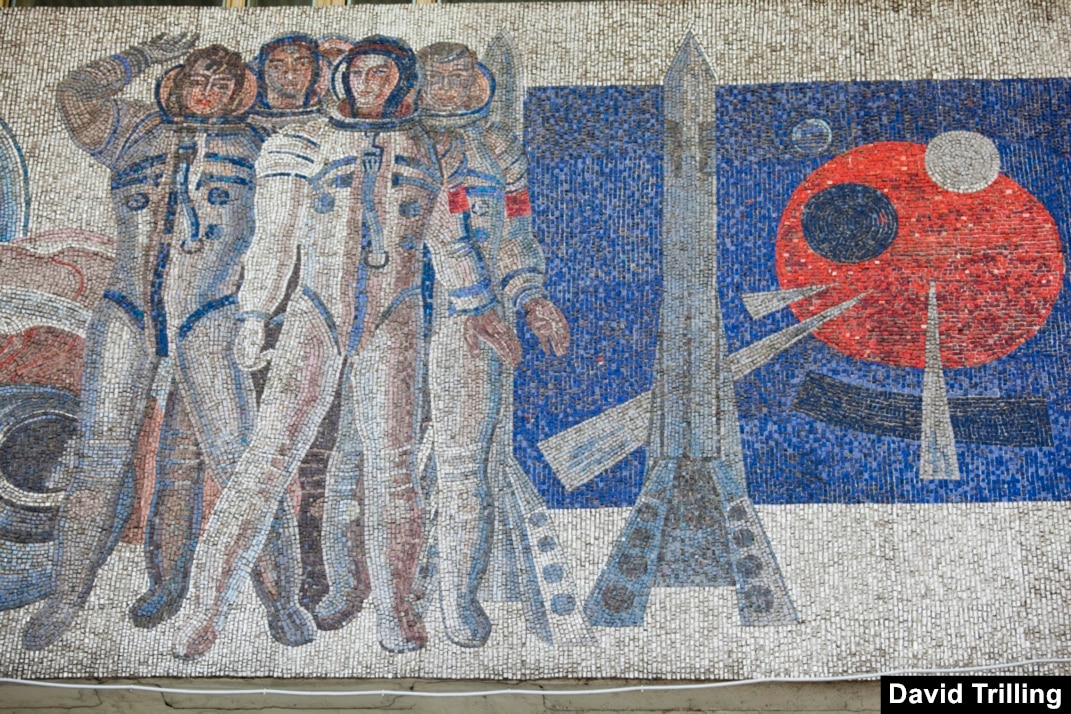This photograph features a striking mosaic artwork, composed of tiny, colorful beads that form a minimalist yet vivid image. The central theme is a space mission, vividly portrayed with four astronauts, each clad in white suits accented with blue lines. The astronauts are positioned on the right side of the mosaic, suggesting they are embarking on an outer space journey. Alongside them, a rocket ship painted in a greyish hue can be seen, poised for liftoff. To the left, there's an enigmatic red circle, reminiscent of a Death Star, set against a contrasting blue background with smaller surrounding circles, adding a layer of intrigue to the scene. This piece merges modern space exploration themes with an aesthetic reminiscent of medieval and Catholic art styles, creating a unique and compelling visual narrative. The artist, David Trilling, has signed his work on the bottom right corner, confirming his authorship of this distinctive art piece.